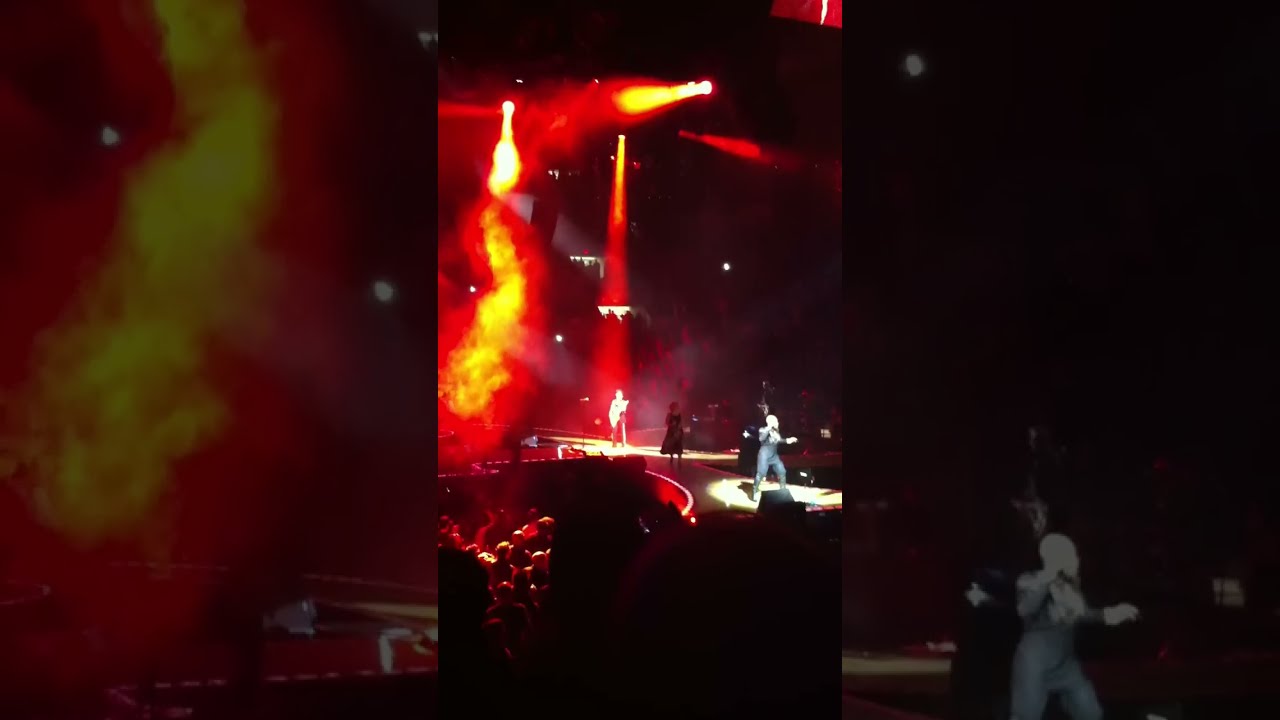The photograph captures a dynamic and atmospheric musical concert. The central focus is a uniquely shaped stage that appears to be inspired by, or actually is, the iconic symbol associated with Prince. The image theme is overwhelmingly red, with deep red lights cascading down from above and casting a saturation that envelops both the stage and the crowd below. Despite the prevailing red, the musicians on stage are distinguished by brilliant white and bright yellow lights. 

On stage, a person, potentially Prince, is seen engaging with the crowd, possibly holding a guitar, while another figure stands to the left. The stage itself contrasts the lighting with its dark, possibly black coloration. Surrounding the stage is a massive, animated audience, creating a sea of energy in the scene. Vertical black strips frame the left and right sides of the image, guiding the viewer's focus towards the center. Above the stage, partially visible at the top, is the bottom edge of a screen likely used to enhance visibility for the concertgoers.